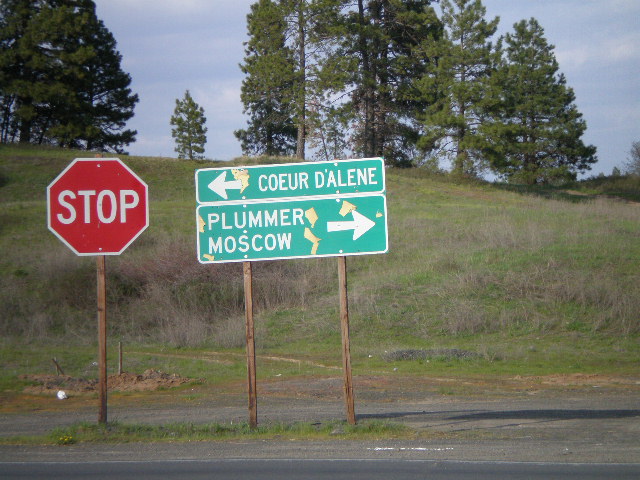The image features a serene outdoor scene capturing the side of a highway under a vibrant blue sky dotted with fluffy white clouds. A line of tall, dark green fir trees form the backdrop, standing atop a gentle, grassy hill that slopes downward. In the foreground, the roadway stretches out, with its edge visible. On the left side of the picture, a prominent red stop sign stands, accompanied by a green and white directional sign. The directional sign features two arrows: one pointing left towards Coeur d'Alene and the other pointing right, indicating the directions to Plummer and Moscow. The entire scene is devoid of people, offering a peaceful and untouched landscape.